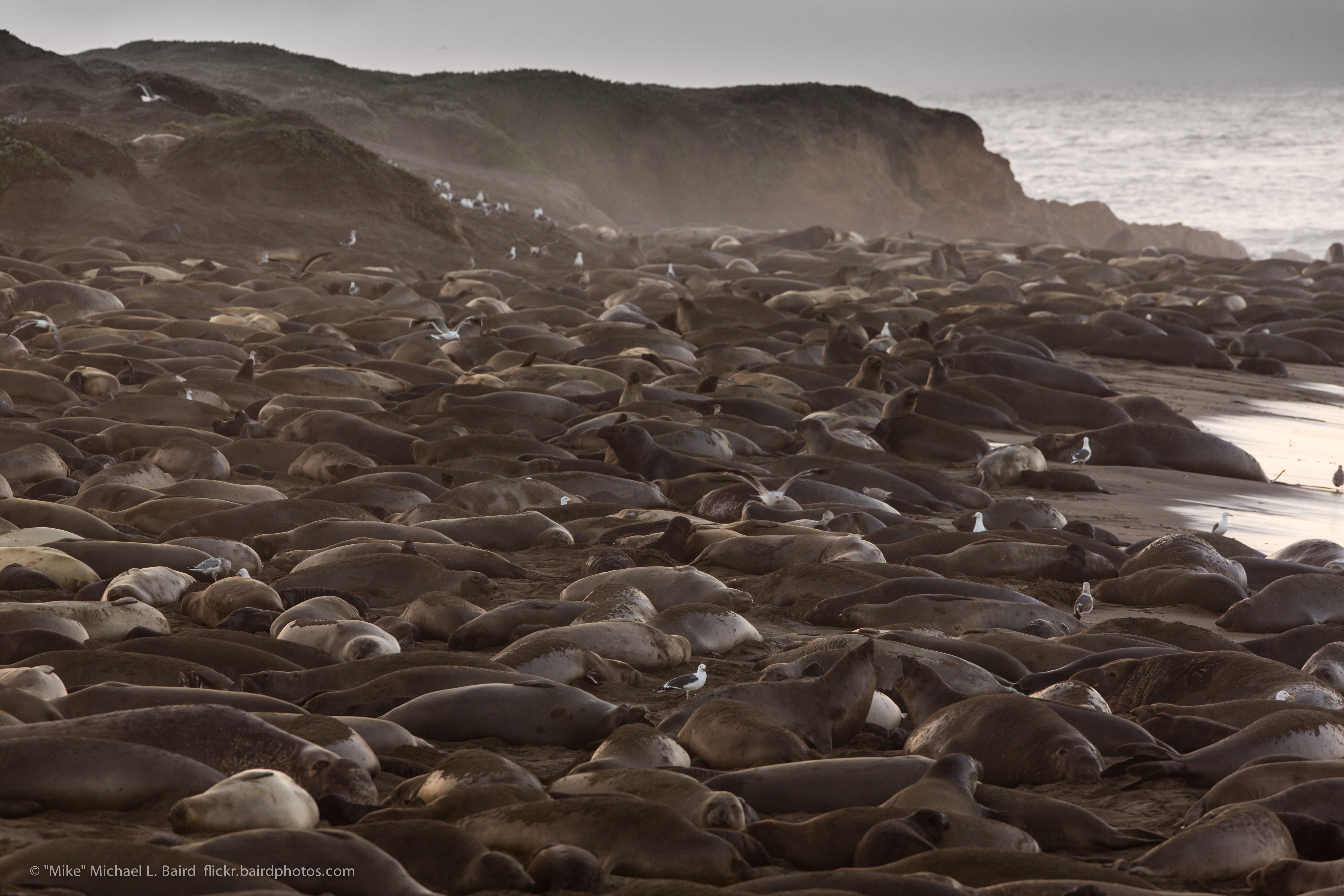In this horizontal, rectangular photograph, a vast expanse of dark brown and black seals or sea lions covers the sandy ground completely, creating a striking visual of wildlife lounging side by side. In the background, the distant ocean stretches beneath a gray sky, which is slightly lighter in the upper left corner. The left side of the image features a rocky, rugged, and small mountainous area that appears scalable. Tiny figures of people are visible, seemingly traversing a trail along this rocky formation. On the right side, patches of sand intermittently peek through, illuminated by streaks of sunlight breaking through the otherwise overcast atmosphere. This vibrant juxtaposition of land, sea, and wildlife is further authenticated by a copyright at the bottom of the image, which reads, "Mike, 'Michael L.'," accompanied by a subtle beard icon.